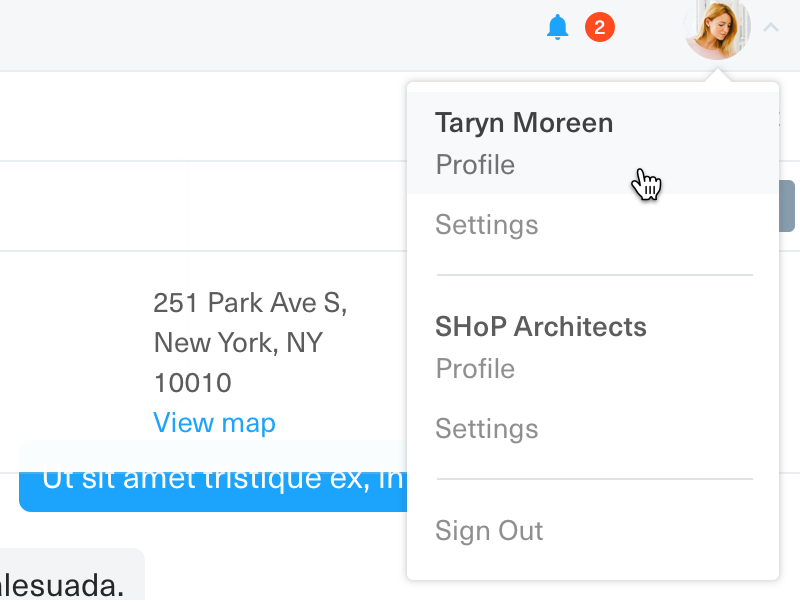A screenshot from a website featuring a predominantly white background with black text. In the upper right corner, there's a circular profile picture of a young white woman with long blonde hair, gazing slightly downwards to her right. Adjacent to her image, there is a red circle displaying the number two and a blue bell icon. The screen captures an active session, suggesting the woman is interacting with the website, as indicated by a pop-up that points to her profile picture and reads "Taryn Maureen profile." A finger emoji directs attention to this area, followed by options labeled "Settings," "Shop Architects Profile," "Profile Settings," and "Sign Out." To the right of this section, a smaller white box provides an address: 251 Park Avenue South, New York, NY 10010, with a clickable "View Map" link in blue. The context implies that either the woman is managing her online profile or someone is searching for information about her on this website.